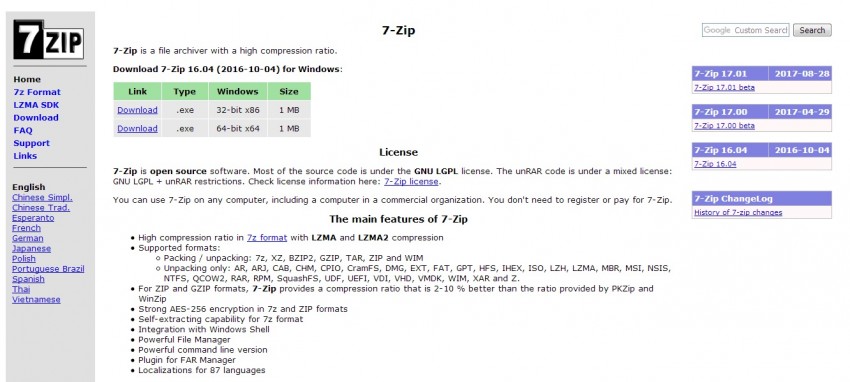The image features a clean white background with the 7-Zip logo prominently displayed. The logo consists of a black rectangle containing the numeral "7" in white, and a white rectangle featuring the word "Zip" in black.

At the top of the image, there is a search bar populated with the text "7-Zip." Adjacent to the search bar is a gray rectangular button containing the word "Search" in black. Below, there is a description that reads, "7-Zip is a file archiver with a high compression ratio."

Further details indicate the availability to download 7-Zip version 16.04, released on October 4, 2016, specifically for Windows. The download section includes two distinct rows each beginning with "Download .exe." The first row is tagged for 32-bit x86 systems with a file size of 1 MB, and the second row is tagged for 64-bit x64 systems, also with a file size of 1 MB.

Additional information notes that "7-Zip" in bold, is open source software, also in bold. The majority of the source code is released under the GNU LGPL license, and the acronym "LGLP" is fully capitalized. 

The main features of 7-Zip are listed in a bullet-point format. On the left side of the image, a navigation menu is visible with links in blue for "Home," "7-Zip," "Format," "LZMA," "SDK," "Download," and "FAQ."